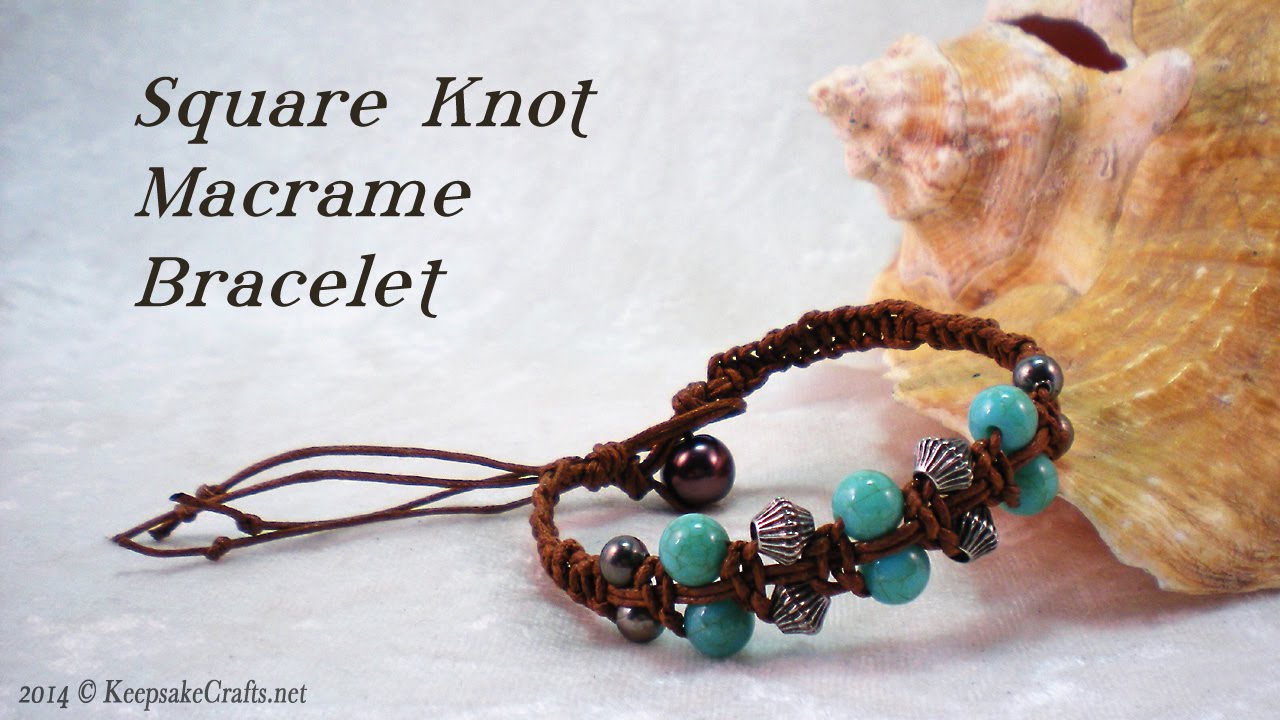The image features a detailed, digitally-created photograph of a brown woven square knot macramé bracelet set against a light blue cloth background. The bracelet, positioned centrally, is adorned with various beads and decorations: a purple spherical bead, two groups of six silver beads, six blue beads, and four uniquely shaped silver beads. The bracelet is draped next to a large seashell that is brown, white, and tan with a noticeable hole. In the top left corner, in black text, is the label "Square Knot Macrame Bracelet," while the bottom left corner features gray text that reads "2014 © KeepsakeCrafts.net." Shadows cast by the items add depth and dimension to the overall presentation.